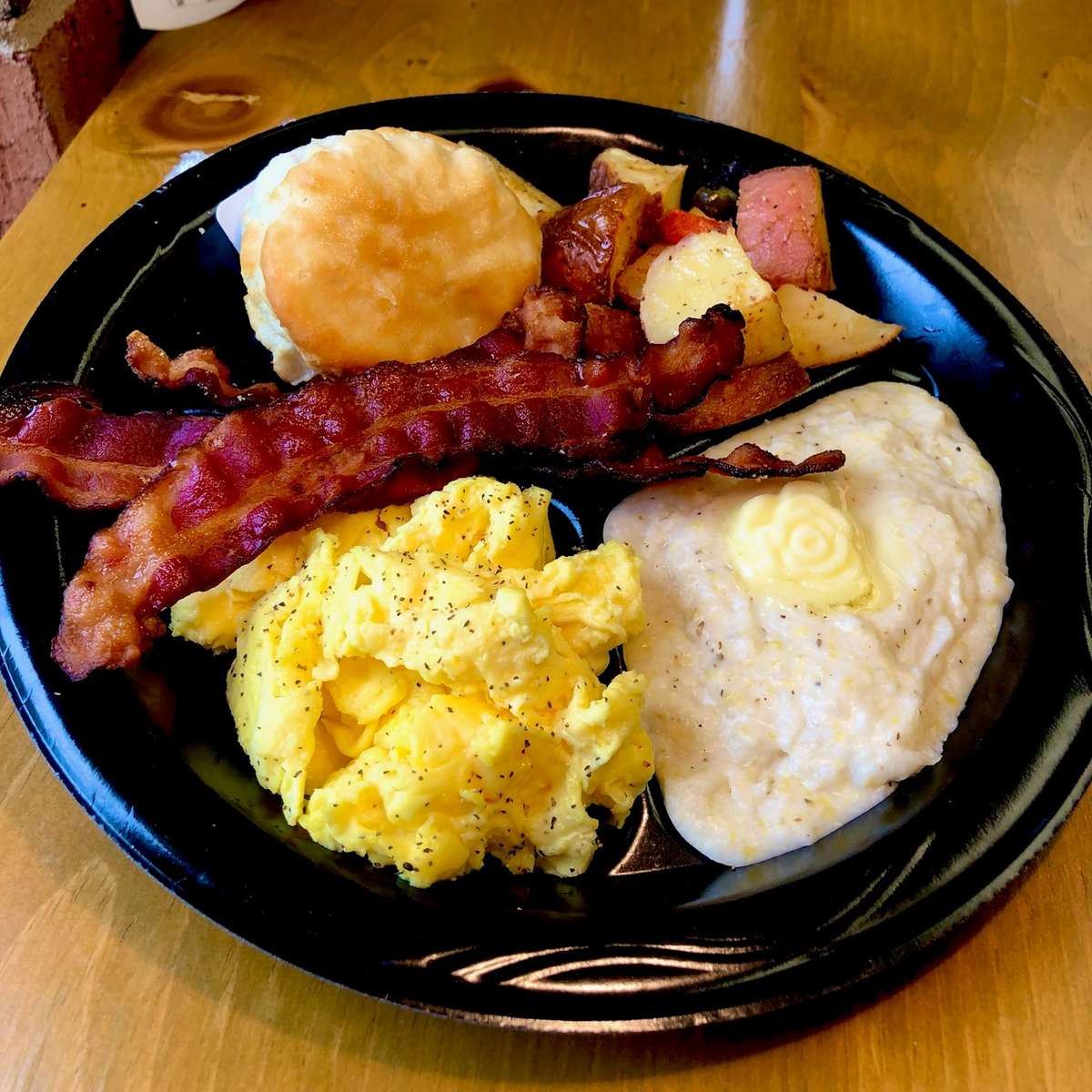In this photograph, a nearly square image captures a detailed breakfast plate positioned on a shiny wooden table with a light brown hue. The plate itself is circular, black, and glossy, featuring various food items meticulously arranged. At the top of the plate sits a large light brown biscuit. Below it, there are several dark red strips of cooked bacon. To the side, you can see a scoop of fluffy yellow scrambled eggs. Adjacent to the eggs is a small pile of hash brown potatoes, showcasing red skins and yellow flesh. Lastly, a portion of white, porridge-like grits, topped with a slightly melted pat of butter, occupies another section of the plate. The different foods are sectioned off on the plate, providing a visually appealing and organized presentation.